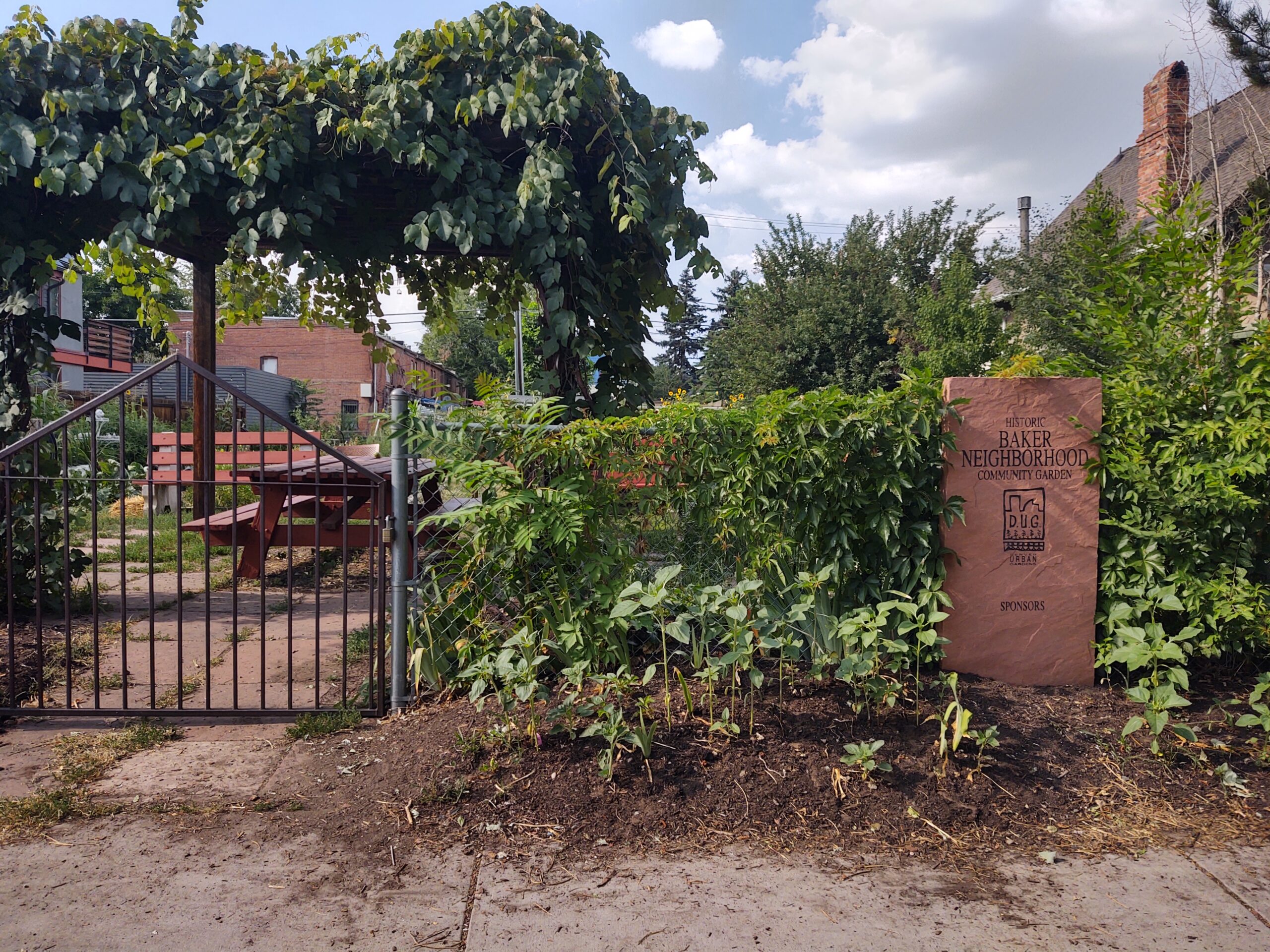This photograph captures a serene and inviting scene of a community garden situated within a residential neighborhood. The focal point is a charming garden environment enclosed by a low brick wall, approximately 2-3 feet high, adorned with various vines and lush greenery. Prominently displayed on the wall is a sign that reads "Baker Neighborhood Community Garden," accompanied by a crude skyline logo and space for sponsors, though none are listed.

In front of the wall, the garden has raised soil beds with a selection of plants and flowers sprouting awkwardly from them. A paved pathway, interspersed with patches of dirt, leads towards a wooden structure within the garden. This wooden area includes a picnic table and is enveloped by verdant plants with abundant, voluptuous green leaves. Just beyond this enclave, there is a sturdy black metal gate and an iron fence with a triangular peak, furthering the garden’s seclusion.

The overhead view features a picturesque blue sky populated with puffy white clouds, enhancing the garden's tranquil atmosphere. In the background, partially obscured by the foliage, are a few houses with visible rooftops and chimney stacks.

Scattered throughout the garden, you can spot additional picnic tables and benches amidst the leafy canopy provided by tall trees, creating a leafy, lush getaway. The chain-link fence, covered in climbing plants, forms another layer of enclosure, ensuring this petite oasis remains a peaceful retreat amidst the suburban setting.